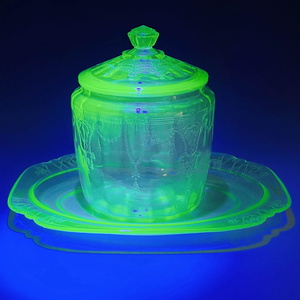The image is a small, detailed photograph that appears to be from an eBay-style listing, showcasing what seems to be antique or vintage Vaseline glassware. The centerpiece is a clear platter with a lidded container resting on it, all of which glow a vibrant green, suggesting it is under a black light, typical of radioactive glassware. The glass is transparent, with a beautiful luminescence that radiates a radioactive-like glow. The setup is placed on a striking metallic blue surface that subtly transitions into a deep black background, creating a visually stunning and collectible item that would appeal to glassware enthusiasts and collectors.